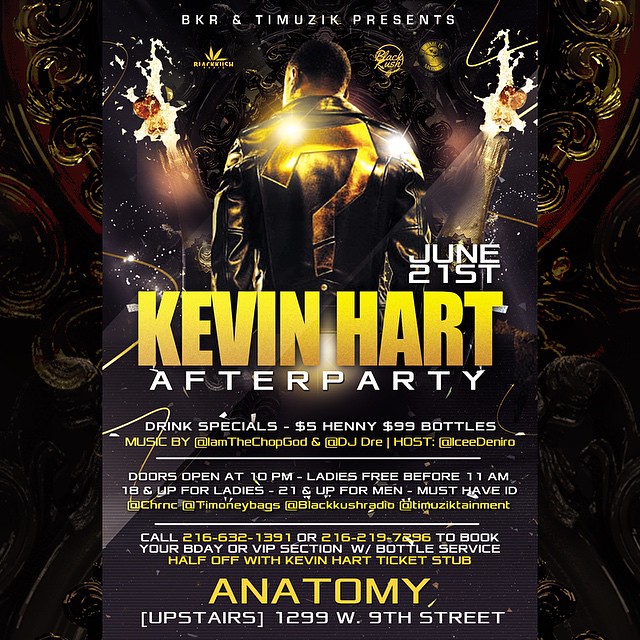This eye-catching advertisement poster for the Anatomy Nightclub prominently features a stylish black man wearing a leather jacket adorned with a gold question mark on the back. Surrounding him are two animated champagne bottles with corks popping off energetically. Above, the event is introduced by "BKR and Tim Music Presents" followed by "June 21st Kevin Hart After-Party."

The central text lists key details: drink specials including $5 Henny shots and $99 bottles, with music performed by DJ Dre and I Am The Chop God. Hosted by Al C. DeNiro, the event promises excitement and exclusivity. The poster highlights that doors open at 10 p.m., and women get free entry before 11 p.m. (likely a typo, suggesting 11 p.m. instead of 11 a.m.), with age restrictions of 18+ for women and 21+ for men. It emphasizes the necessity of ID for entry.

Additional information includes booking phone numbers for VIP sections or birthday reservations. Those with a Kevin Hart ticket stub receive half off the bottle service. The venue is identified as Anatomy, located at 1299 West 9th Street. The vibrant border, featuring red, gold, and black designs, encapsulates the poster, enhancing its visually dynamic appeal.